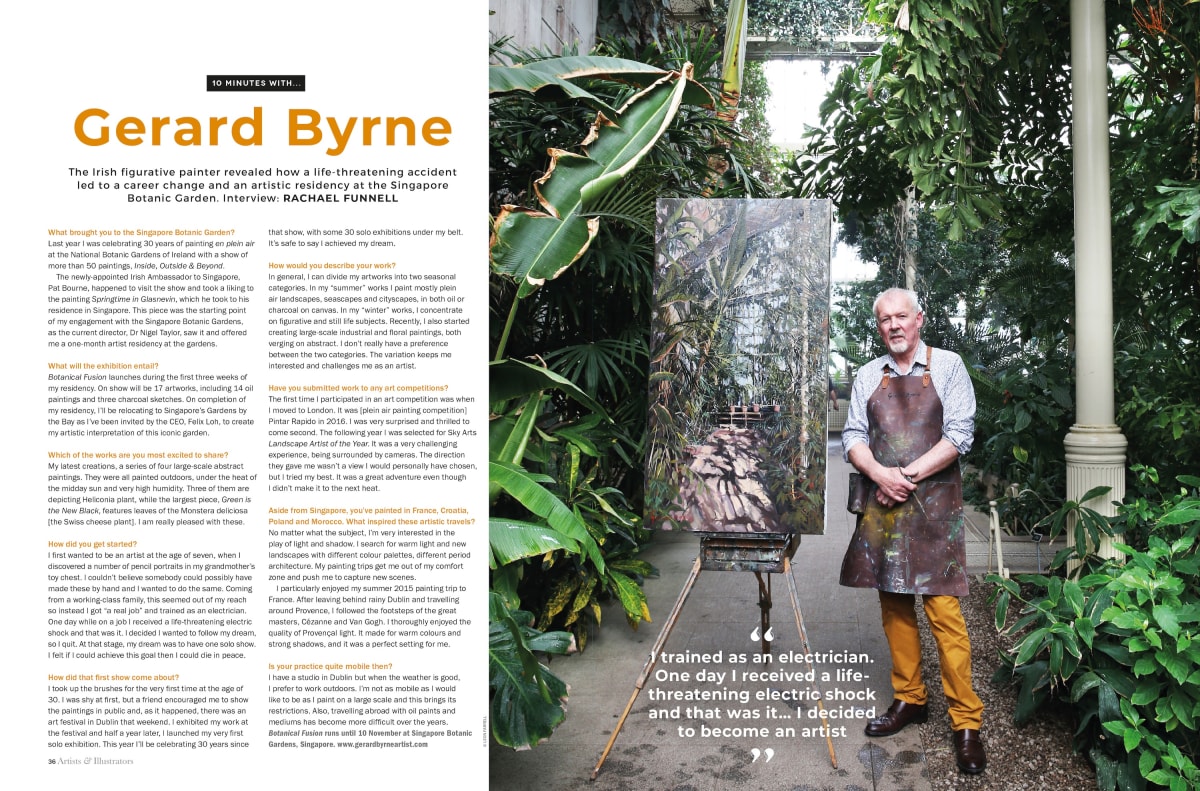In this captivating image, we see renowned Irish figurative painter Gerard Byrne, who transitioned to an artistic career following a life-threatening electric shock. He stands on a cement walkway flanked by lush greenery in the Singapore Botanical Garden, where he is participating in an artistic residency. Byrne is dressed in a blue long-sleeve shirt, a paint-splotched leather apron, tan-colored pants, and dress shoes. He poses with his hands crossed over his belly beside one of his stunning nature paintings set on an easel, depicting a forest path with an intriguing bridge in the distance. The scene is lit by a nearby lamp post, adding to the serene, natural atmosphere of the garden that serves as both his inspiration and workplace.